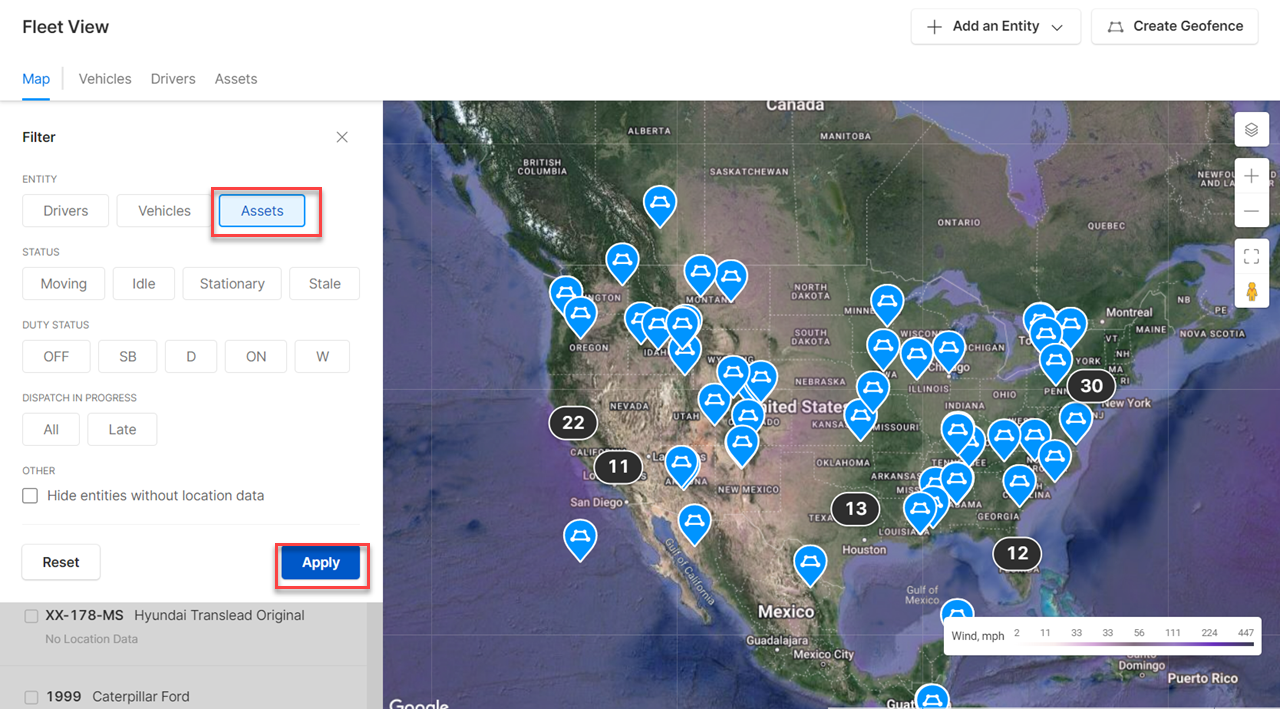The image displays a detailed map of the continental United States, extending slightly into Canada and Mexico. The map is populated with numerous blue markers, which presumably represent semi-trucks. The map itself is rendered in a terrain-like view, illustrating the flatlands of the Midwest, the varied elevations of the East, and the distinct topography of the West Coast.

On the left side of the image, there is a filtering interface featuring options such as drivers, vehicles, and assets, with the 'assets' filter highlighted by a box. The interface also allows filtering by the status of the trucks—whether they are moving, idle, stationary, or stale—although none of these options have been selected. Additional filters include duty status with acronyms like S-B-D-O-N-W that are not explicitly explained, and options for dispatch in progress and hiding entities within a specific location unit.

At the bottom right of this pane, there is a blue "Apply" button. The overall setup appears to be a sophisticated system for tracking the location and status of freight and trucks across the map.